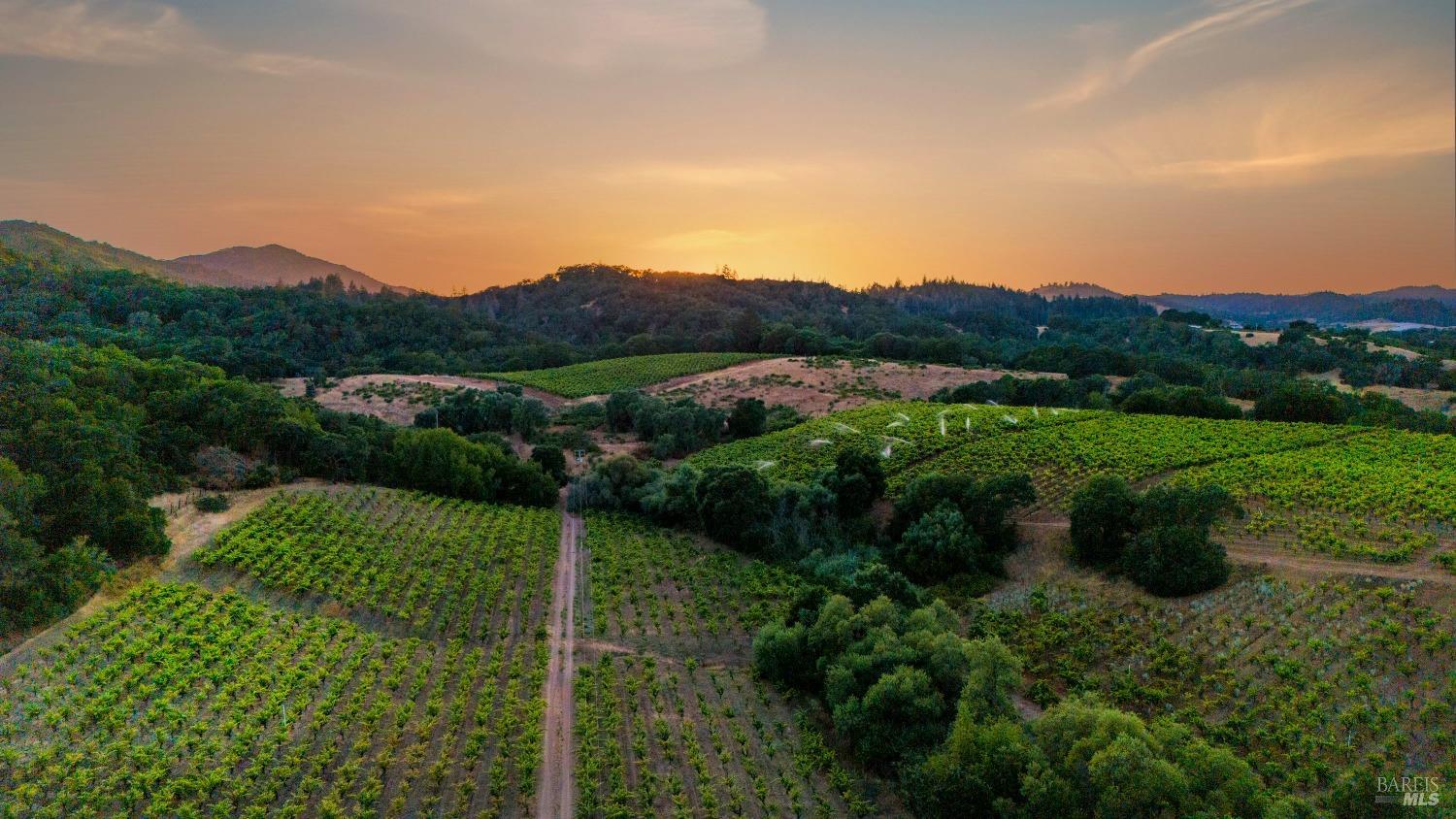This photograph showcases a sprawling expanse of farmland under a vibrant sunset, with hues of orange and gold illuminating the horizon. Dominating the left side of the image is a majestic mountainscape, while thick forests and brush frame the farmland from all sides. The aerial perspective offers a comprehensive view of the well-organized plots of agriculture, featuring rows upon rows of lush green crops. Some plots are being actively irrigated by visible sprinklers. A narrow road winds through the middle of the fields, providing access to the various sections of the farm. In the right-hand corner of the image, a small body of water nestles against the backdrop of rolling hills and dense trees. The entire scene is bathed in the soft glow of the setting sun, creating a picturesque and serene agricultural landscape.